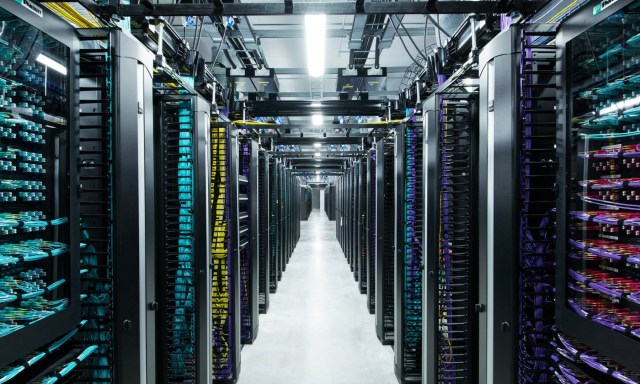The image depicts an industrial-scale server room with a long, narrow hallway lined with towering server racks on both sides. The environment is meticulously clean, featuring a pristine white floor and metallic gray, silver walls. The racks are filled with an array of computer equipment, each adorned with vibrant colored lights and wiring. The left side displays green wiring and lights, while the right side showcases an assortment of purple and green, complemented by occasional red indicators. Small sections of yellow wiring are visible, leading from some partitions toward the ceiling. Fluorescent lights illuminate the space from above, enhancing the visibility of the intricate technical details. The scene is devoid of people and text, emphasizing the high-tech and organized nature of the server room. The overall ambiance is one of advanced technology with elements like glass doors on high-tech refrigerators, revealing a colorful and illuminated interior.